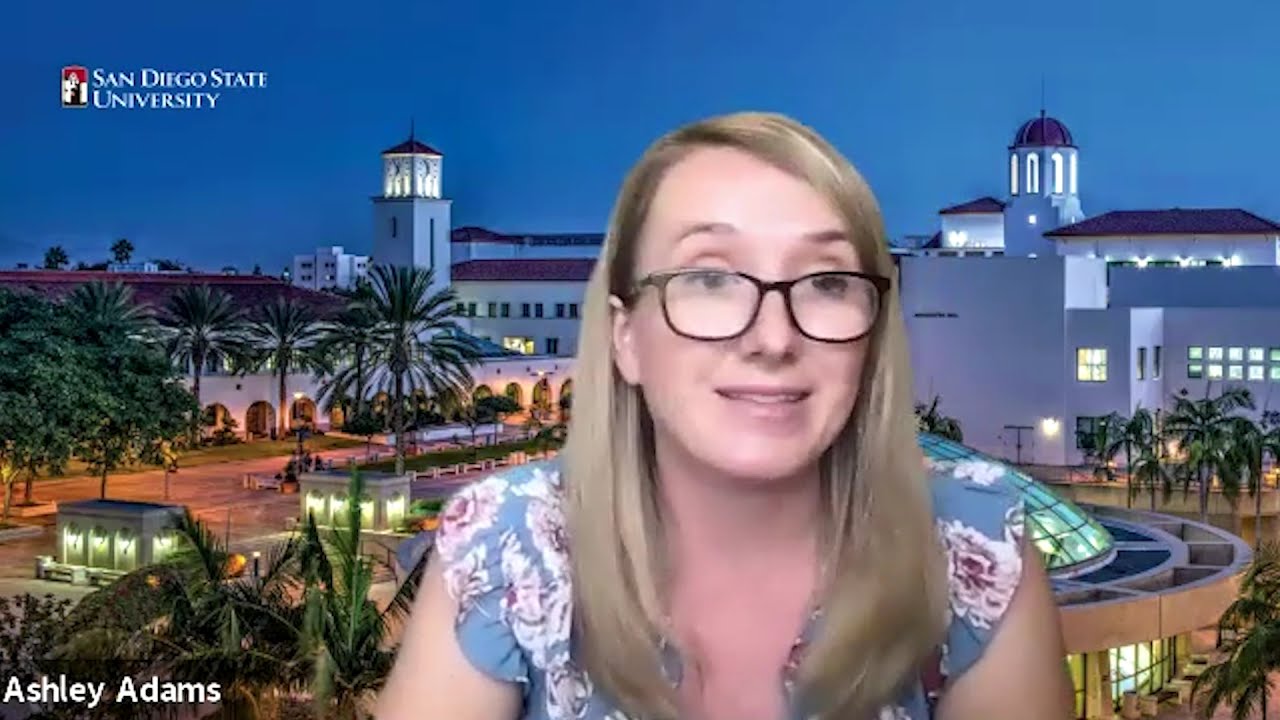This is a color photograph featuring a young Caucasian woman, likely in her early 20s, positioned in the upper left-hand corner. Her shoulder-length blonde hair complements her brown-rimmed glasses, which sit slightly down her nose, aligning the top rim with her eyes. She gazes slightly off to the viewer's right with her eyebrows raised, her mouth partially open to reveal her teeth, suggesting a mid-smile. She wears a short-sleeved blue blouse adorned with large pink and white floral patterns and subtle ruffle details.

In the background, there appears to be a superimposed image of San Diego State University's campus, characterized by its distinct Spanish-style, mission-style architecture. The buildings are prominent with their white adobe walls and red terra-cotta roofs, accompanied by illuminated towers. The scene is set during dusk, casting a soft light upon the campus plaza, which is populated with palm and other trees. In the upper left corner of the photograph, there's white text displaying “San Diego State University” alongside the university's logo. The lower left corner bears the name "Ashley Adams" in the same white text, presumably identifying the woman in the photograph.